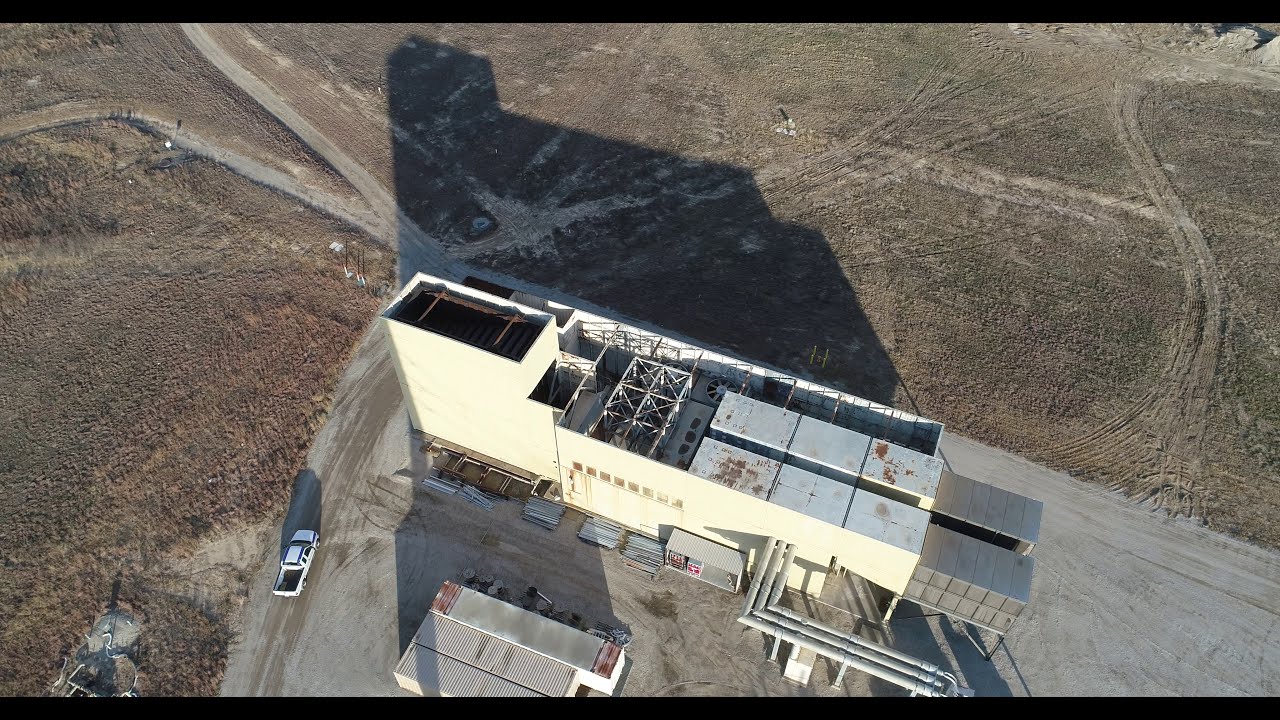This aerial photograph depicts a large, predominantly white and tan industrial building, likely a factory or manufacturing plant, situated in a desolate and undeveloped area that resembles a desert environment, similar to scenes from the movie "Oppenheimer." The surrounding landscape is stark and barren, characterized by flat, expansive tracts of brown, greenish, and reddish ground with no houses, trees, or significant infrastructure. Visible pathways suggest access routes for vehicles, with a notable pickup truck seen heading towards the building from the lower left. The building is shadowed towards the upper part of the image, and multiple containers and several horizontal black strips are present at the top and bottom edges of the photograph. Additionally, three prominent pipes extend perpendicularly from the building, indicating potential industrial activities.